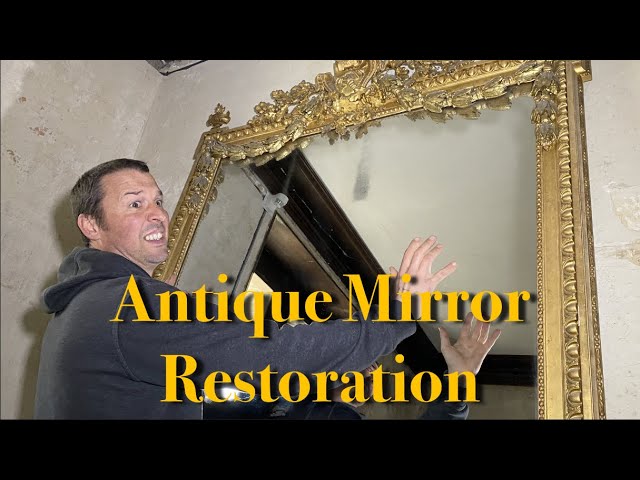The image depicts a man with brown hair and a surprised expression on his face, reaching for a large, antique mirror with a gold, intricately-carved frame. He's dressed in a gray hoodie and is captured in mid-action with his hand touching the mirror, reflecting his hands and hinting at the beginning of a restoration project. The background consists of off-white, slightly damaged walls. Superimposed in yellow text, the caption reads "Antique Mirror Restoration," indicating a screenshot possibly from a video. The man's open-mouthed expression conveys either concern or focus on the task ahead.